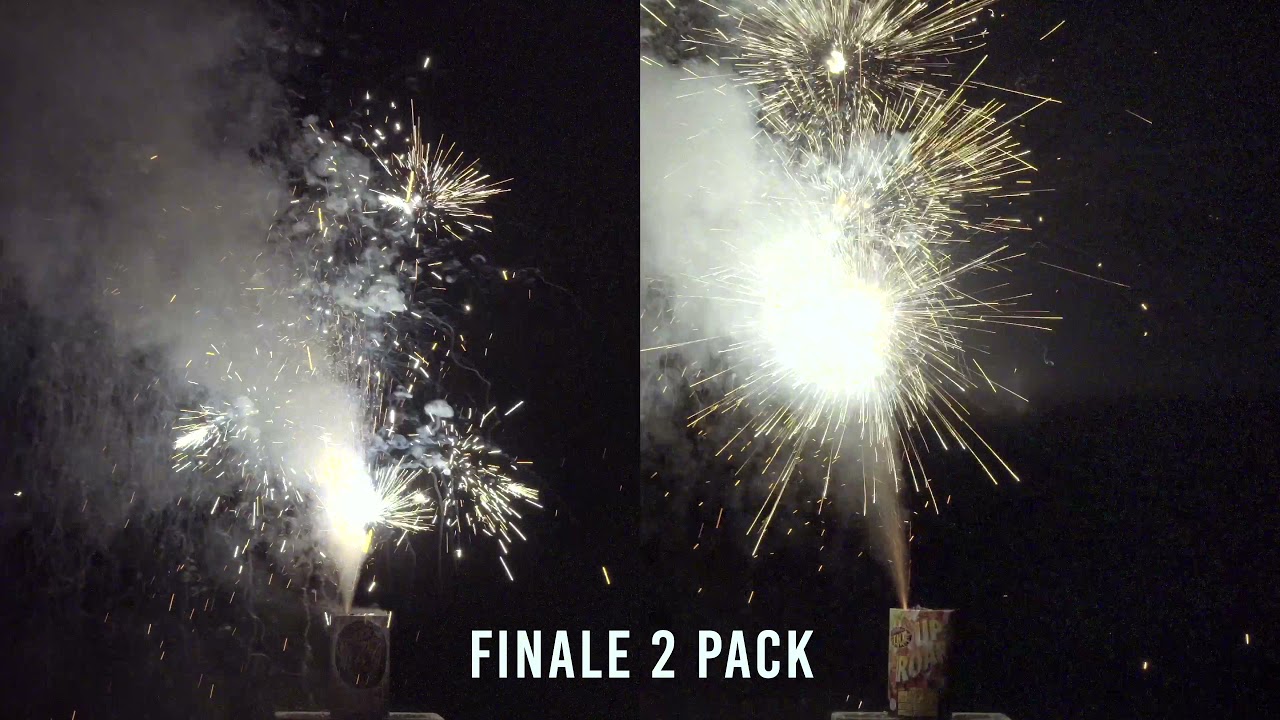A horizontally oriented rectangular collage features two nighttime photographs of fireworks against a black background, likely part of an advertisement. Centered at the bottom of the image, bold white text reads "FINALE 2-PACK." In the left photograph, a small, colorful canister, partially visible at the bottom, emits bright white and yellowish sparks amidst thick, dark smoke. The right photograph offers a closer view of a similar canister, revealing some of the lettering on it, including the word "UPROAR." This canister shoots higher, producing a more dramatic display with whiter smoke and more intense yellow sparks. Both images capture the vibrant, dynamic shimmer of the fireworks, highlighting their vibrant bursts and trails of light.